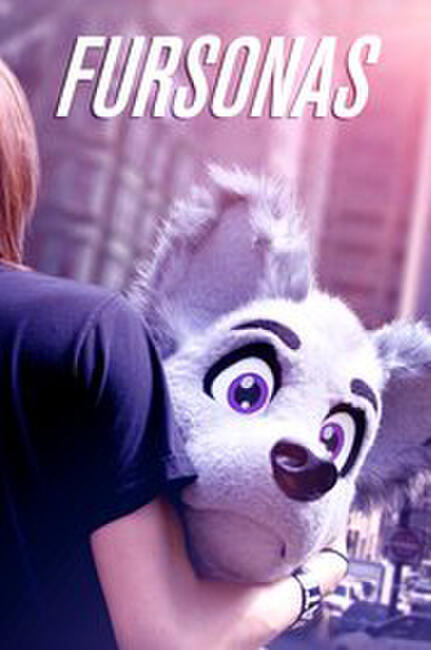In this faintly colored image dominated by shades of purple and light lavender, a person wearing a dark blue t-shirt—possibly with a purplish hue—holds a large stuffed animal head. The person's brownish-red hair and partial appearance on the left side of the image add to the intriguing composition. The stuffed animal, resembling a cartoon dog with big fluffy ears, notable white fur, purple eyes, and a large black nose, looks concerned or surprised, its eyes wide and expressive. Adding to the scene, the person holding the stuffed dog has a black wristband or watch on their right wrist. The backdrop features blurred tall buildings, suggesting an urban setting, while the top of the image prominently displays the text "FURSONAS" in capital letters, possibly indicating a brand or theme.